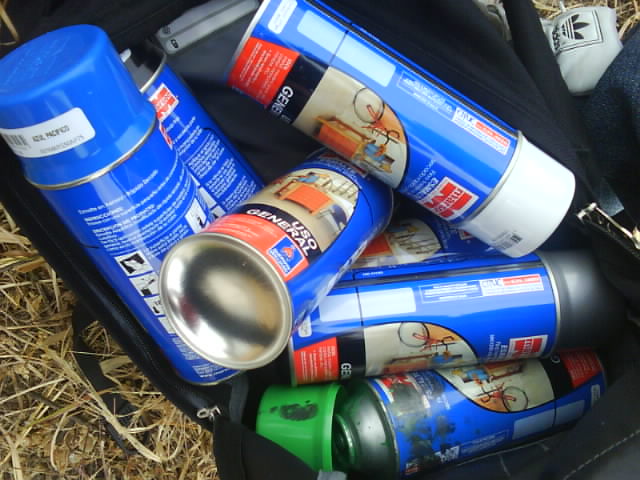In this detailed image, we see a disorganized pile of spray paint cans inside a black bag, which suggests it might be used as a graffiti artist's kit. The cans are predominantly blue, with various lid colors including green, white, blue, and orange, indicating a wide array of paint colors such as silver, green, white, black, and blue. One of the cans has spilled gray or silver paint. The bag, which resembles a piece of luggage or a large backpack with visible zippers, lies on a patch of burnt-out grass or hay, giving a light brown and string-like texture to the ground. In the top right-hand corner, there's a white item of clothing or possibly a shoe featuring the black-and-white Adidas logo. Additionally, there's a white Adidas tennis shoe slightly visible under the bag, emphasizing the haphazard nature of this scene. The bag is open, showcasing the spray cans inside, and the overall setup suggests mobility and quick access, ideal for a graffiti artist who might need to move swiftly. The image captures a messy yet functional arrangement ready for swift use.